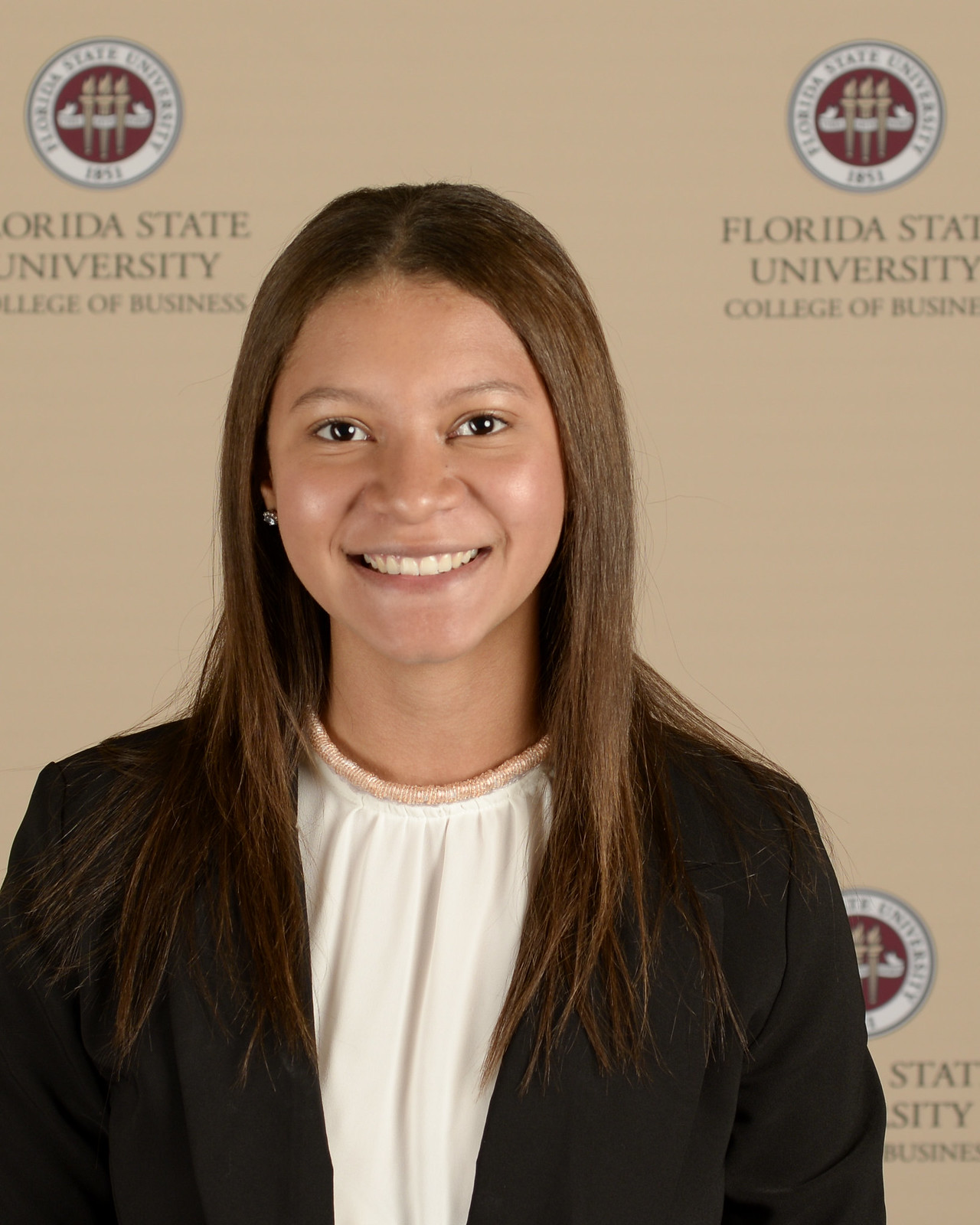The photograph features a smiling young woman, likely of college age, with long, straight brown hair that extends beyond her shoulders. She has a medium-light complexion and a pleasant smile revealing nice teeth. She is adorned with small, gem-studded earrings in her ears and a peach-colored beaded necklace that lies just above the collar of her white blouse. Over her white blouse, she wears an open black business coat. The backdrop is a solid tan color, featuring a repeated logo of Florida State University College of Business. The logo includes a prominent circle with three torches within it. The image captures a professional yet warm and approachable demeanor, highlighting her as a representative or student of the college.